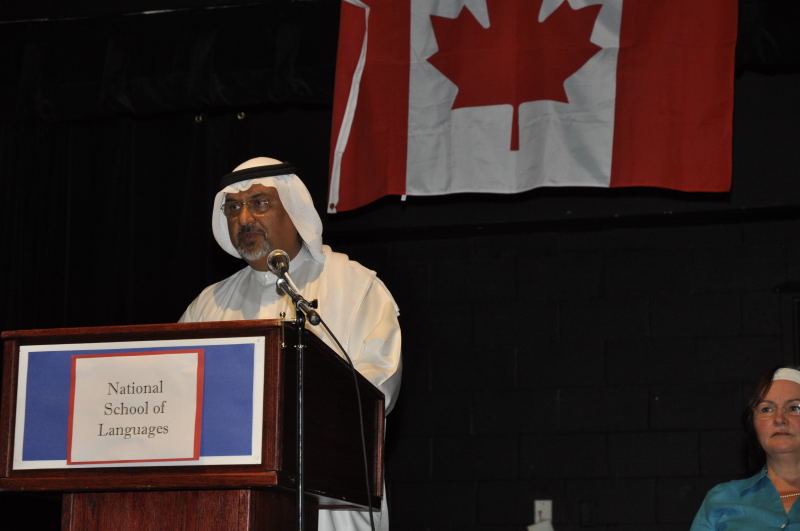In this photograph, a man of Middle Eastern descent, identifiable by his brown skin and traditional attire, stands on a dimly-lit stage. He is wearing a white headdress with a black band and a floor-length white tunic. He has a grey goatee, glasses, and appears somewhat annoyed, looking off-stage. The man is speaking into a microphone attached to a dark wood podium, which prominently features a blue sign with the text "National School of Languages" on it. Behind him, a large Canadian flag is prominently displayed on the wall. To the lower right of the podium sits a middle-aged white woman with dark brown hair tied back in a white headband. She wears glasses, a light teal blue collared button-up shirt, and pearls, and has a grim expression on her face. The overall lighting of the image is quite dim, with a visible plug in the background adding to the indoor setting’s ambiance.